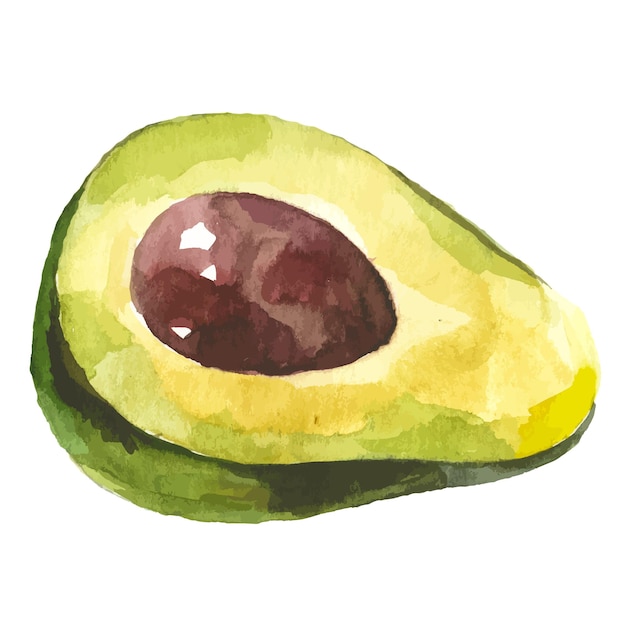This image features a detailed watercolor painting of a neatly sliced half avocado set against a stark white background. The realistic depiction showcases the avocado's dark green outer peel transitioning into a lighter green around the edges, suggesting a natural reflection. The fruit’s flesh is illustrated in varying shades of light lime green, yellow, and green, capturing the gradient typical of a ripe avocado. At the center, the prominently displayed pit is painted in shades of brown with subtle white highlights, giving it a reflective quality that indicates the light source. The shadows and white spots around the pit enhance the realistic texture of the avocado. The careful, gentle brush strokes lend a delicate touch to the overall composition, making it appear as though it could be a piece taken from an artist's portfolio.